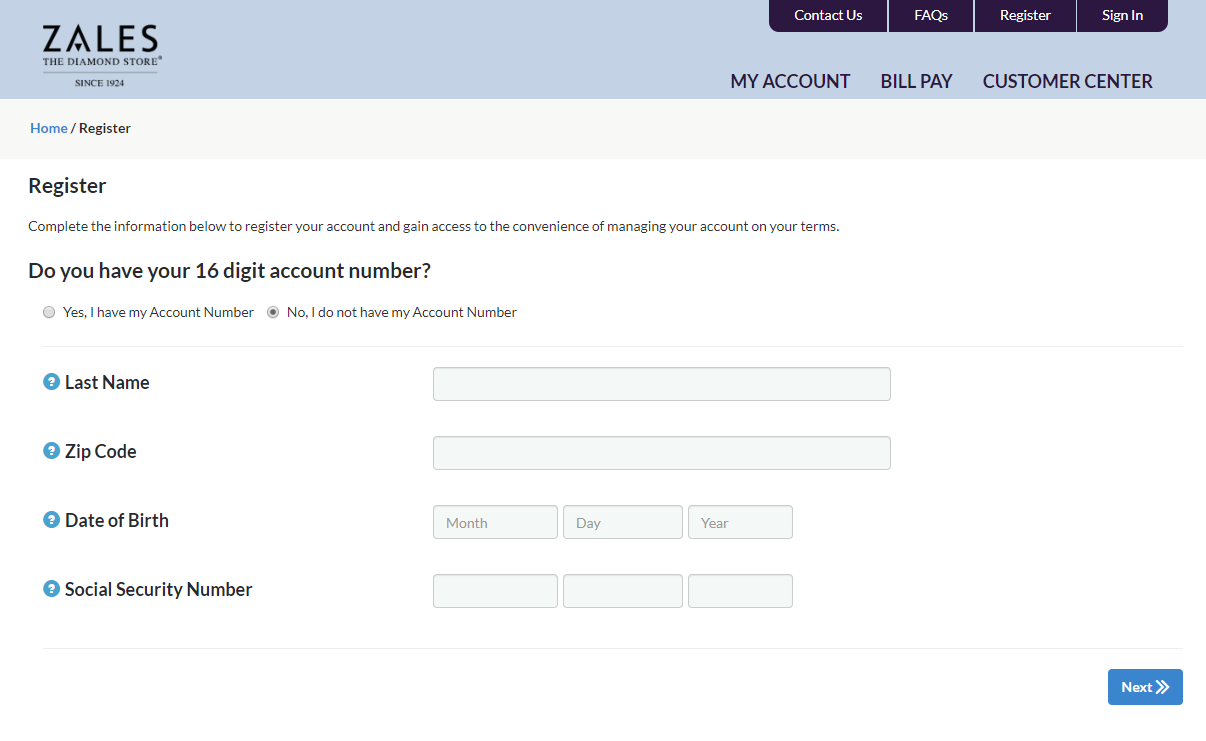The image is a detailed horizontal screenshot of the Zales store's registration webpage. At the top left corner, the Zales logo is prominently displayed, featuring the characteristic Zales lettering with an arrow at the bottom of the 'A'. Below the logo, it states, "Zales, The Diamond Store Since 1924."

The upper part of the image features a blue-gray banner with navigation options, including 'Contact Us,' 'FAQs,' 'Register,' and 'Sign In,' located on the right side. Additionally, there are links for 'My Account,' 'Bill Pay,' and 'Customer Center' below these options.

The main section of the webpage, titled 'Home / Register,' is situated under the top banner. 'Home' is clickable and styled in blue text, allowing users to return to the homepage easily.

The registration section prompts users to indicate whether they possess a 16-digit account number, with options to select 'Yes' or 'No.' On the left side, text boxes are provided for entering the 'Last Name,' 'ZIP Code,' 'Date of Birth,' and 'Social Security Number.' The 'Date of Birth' entry is divided into three separate fields for the month, day, and year. Similarly, the 'Social Security Number' is segmented into three fields to match the number format.

A blue dot featuring a question mark is positioned to the left of the input list, likely indicating additional information or help. The layout has a plain white background without any borders on the left, bottom, and right-hand sides of the image. Completing the form is facilitated by a blue 'Next' button located at the bottom right corner.

Overall, the registration page is designed with a clean and minimalistic aesthetic, emphasizing the form fields and navigation options against a simple, uncluttered background.